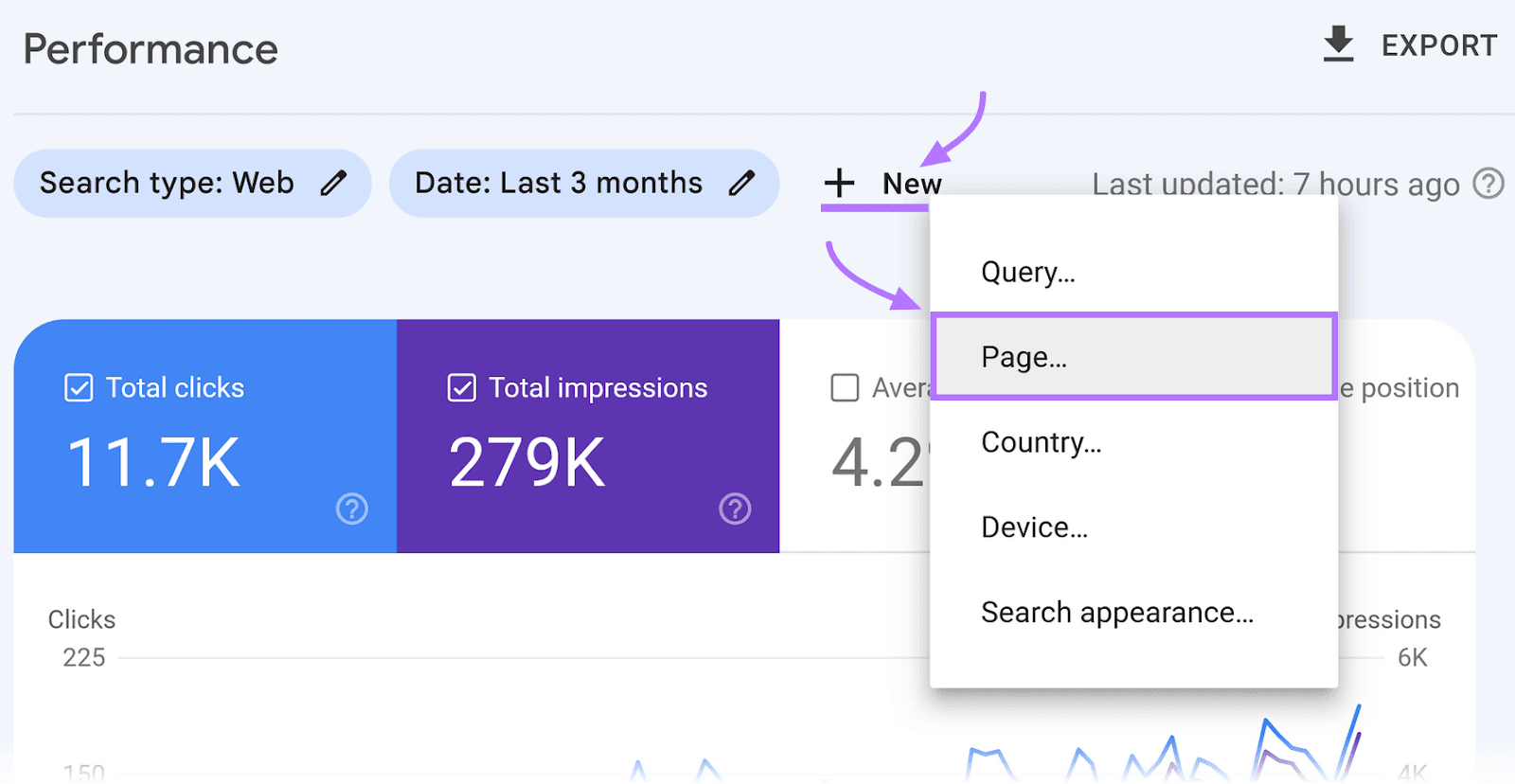A screenshot displays an older YouTube performance page, potentially from Twitch, distinguished by its vintage interface. In the upper left corner, the word "Performance" is prominently featured, while on the upper right, there is a "Download" button accompanied by an "Export" option. Below this, a text line instructs users to "Search the web with a pencil" within a light blue oval outlined with black lettering. Beneath it, another line presents a date filter set to the "Last three months."

Adjacent to these lines, two blue-purple arrows direct the viewer’s attention. The first arrow points to a "Plus New" button highlighted in purple. The second arrow points downwards to a submenu encapsulated in a purple square. This submenu houses options such as "Query," "Page," "County," "Device," "Country," and "Search Appearance."

To the upper left and right portions of the interface, additional metrics such as "Last updated 7 hours ago,” “Total Clicks: 11.7K,” are visible with a checked mark, and “Total Impressions: 279,000.” Below these figures, a partially visible graph tracks various performance metrics including clicks, impressions, and views, providing insight into content engagement, presumably for YouTube or Twitch.